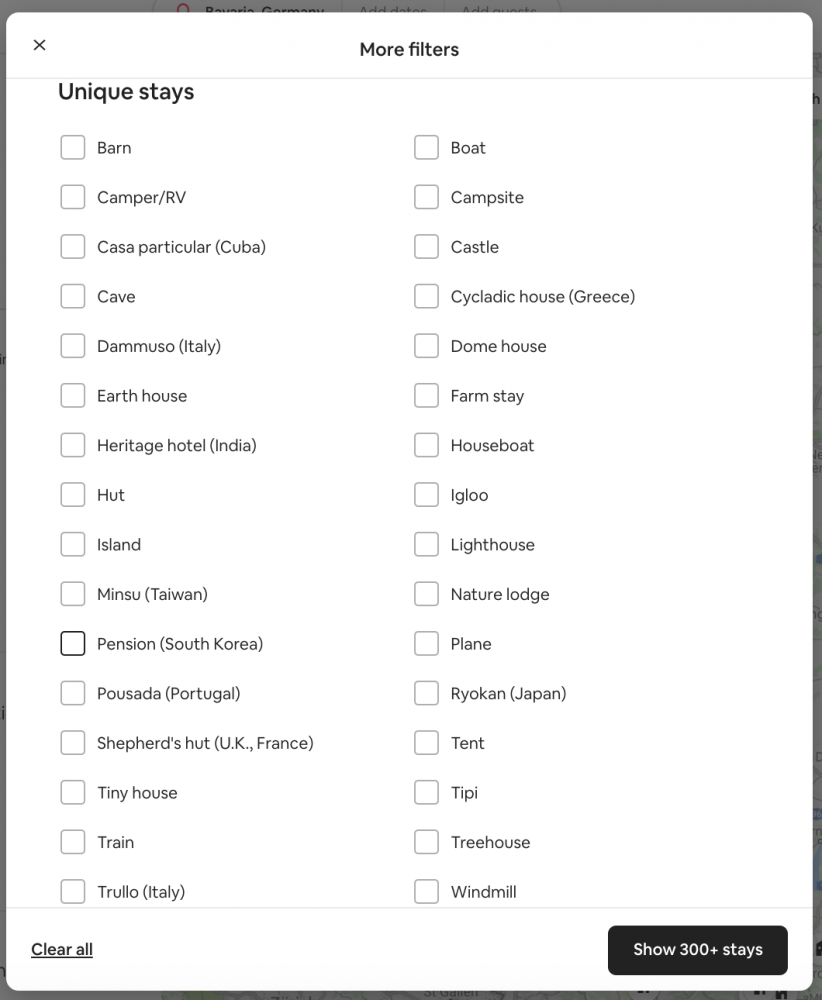This image depicts a vertically-oriented, elongated white rectangle framed by a thin black border, presenting a comprehensive list under the heading "More Filters." The list categorizes distinct accommodation types under the "Unique Stays" section, including:

- Barn
- Boat
- Camper/RV
- Campsite
- Casa Particular (Cuba)
- Castle
- Cave
- Cycladic House (Greece)
- Damuso (Italy)
- Dome House
- Earth House
- Farm Stay
- Heritage Hotel (India)
- Houseboat
- Hut
- Igloo
- Island
- Lighthouse
- Minsu (Taiwan)
- Nature Lodge
- Pension (South Korea)
- Plane
- Pusada (Portugal)
- Ryokan (Japan)
- Shepherd's Hut (UK, France)
- Tent
- Tiny House
- Teepee
- Train
- Tree House
- Truio (Italy)
- Windmill

Each accommodation option is accompanied by an unchecked checkbox to its left. Immediately below the list, the phrase "Clear All" is prominently displayed. In the bottom right corner, a black rectangle with white text that reads "Show 300+ Stays" invites further action. The overall image notably maintains a taller-than-wide aspect ratio.